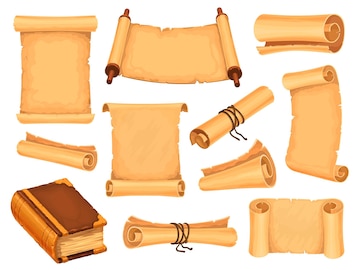The image is a detailed drawing set against a white background, showcasing a collection of varied scroll illustrations, predominantly tan in color. There are 11 distinct scrolls, some rolled up tightly, others loosely, and a few are unrolled. Several scrolls are tied with string, while others are secured with leather thongs. Notably, one scroll toward the top-middle features rollers at both ends, stretching it out. Other scrolls are either open or scrolled in various configurations, some rolled at both ends, some just at one. Among the scrolls, there is a thick brown book located in the bottom left corner, distinguished from the scrolls by its solid form and closed state. None of the scrolls contain any visible text or markings.